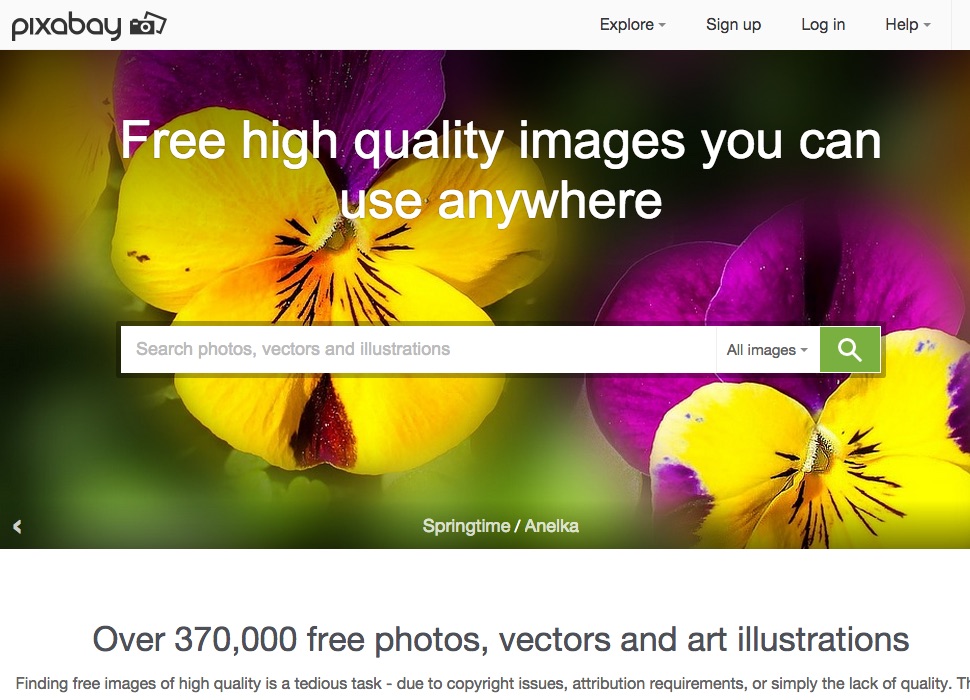This is a screenshot of the Pixabay website, a platform known for providing free photographs and illustrations. The page is dominated by a vibrant, eye-catching rectangular image featuring bright purple and yellow flowers, with two flowers of each color. Overlaying this floral backdrop is white text proclaiming, "Free high-quality images you can use anywhere."

At the very top of the website, on the left side, the word "Pixabay" is displayed alongside a small camera icon, clearly representing the brand. To the right of the logo, there are navigation options labeled "Explore," "Sign up," "Log in," and "Help."

Just below the main banner image, a search bar stands prominently. Inside the search bar, greyed-out placeholder text reads "Search photos, vectors, and illustrations." Adjacent to the search bar, a dropdown menu allows users to filter search results to "All Images," and a green button with a white search icon invites users to initiate their search.

Below the search bar, within the same rectangular image, the text "springtime / Anelika" is noted, likely crediting the photographer or artist. At the very bottom of the image, comprehensive text states there are "over 370,000 free photos, vectors, and art illustrations" available on the site. An additional description emphasizes the challenge of finding high-quality, free images due to various issues like copyright constraints, attribution requirements, and quality standards.